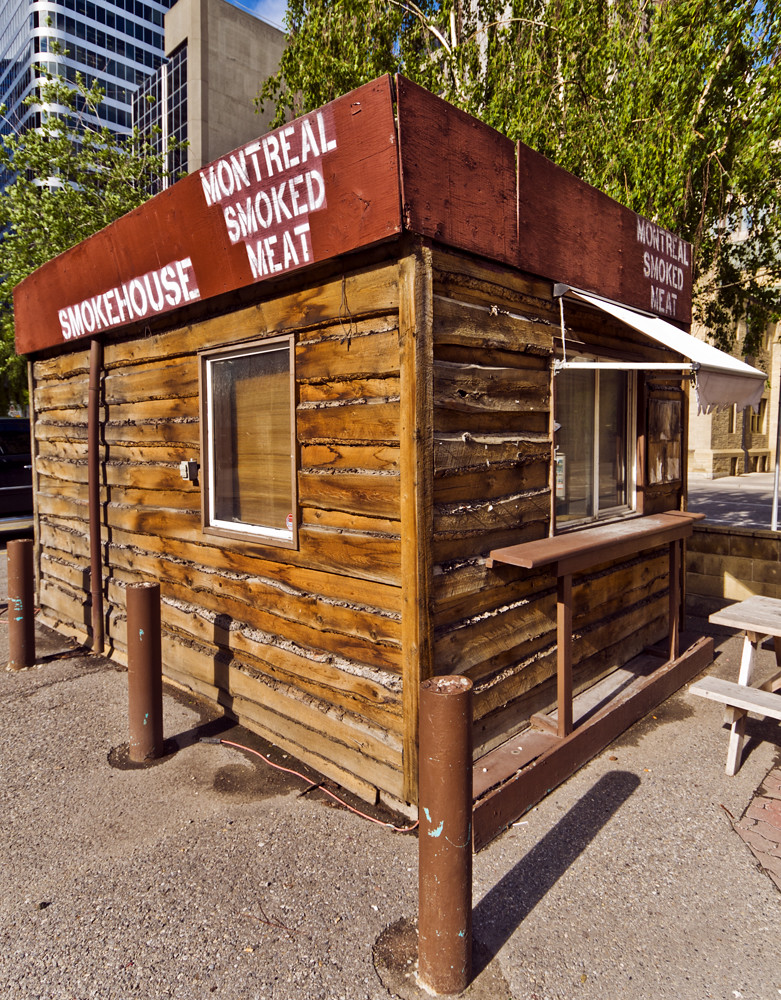The photograph, taken outdoors on a clear day, showcases a small, rustic smokehouse constructed entirely out of varnished timber, exuding a warm, rich brown hue that resembles old-style wood cabin construction. This tiny wooden shack, set against an urban backdrop with paved streets, is neatly boxed in by three cement poles on the ground to its left and a short brick wall that partially disappears behind it on the right. The front of the smokehouse features a closed sliding window accented with a small white awning and a shelf, primarily designated for ordering and receiving food. Above this window and on the left side atop the front panel, bold white stencil letters spell out "Smokehouse, Montreal Smoked Meat." Another identical stencil is visible on the right side of the front. Adjacent to the window, there appears to be a menu. A wooden table with small benches is partially visible in front of the shack, hinting at a picnic-style dining arrangement. The entire scene suggests a quaint, inviting setup for enjoying Montreal smoked meat, surrounded by subtle urban elements.